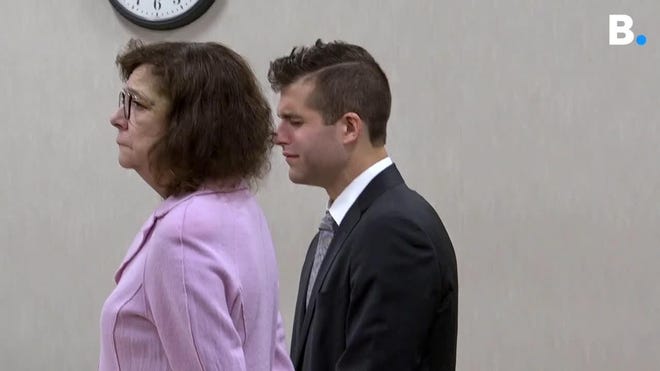In this image, we see a poignant courtroom scene set against a drab, gray-beige background. In the top right corner, there's a prominent, bold white letter "B" set against a blue circle. To the upper left, the bottom portion of a round clock with a black frame is visible, showing the number six.

At the center of the image stands a Caucasian woman in her 50s, wearing glasses and a lavender blazer. Her short, frizzy, dark brown hair contrasts with the somber atmosphere. The woman's hands are seemingly behind her back, and she exudes an air of concern and solemnity.

Directly behind her is a younger Caucasian man who appears deeply distressed, possibly crying. His hair is shaved on the sides and styled into a short mohawk. He is dressed formally in a black suit, a white collared shirt, and a gray tie. The serious mood and their shared sorrow suggest they are actively engaged in an ongoing trial or court case.